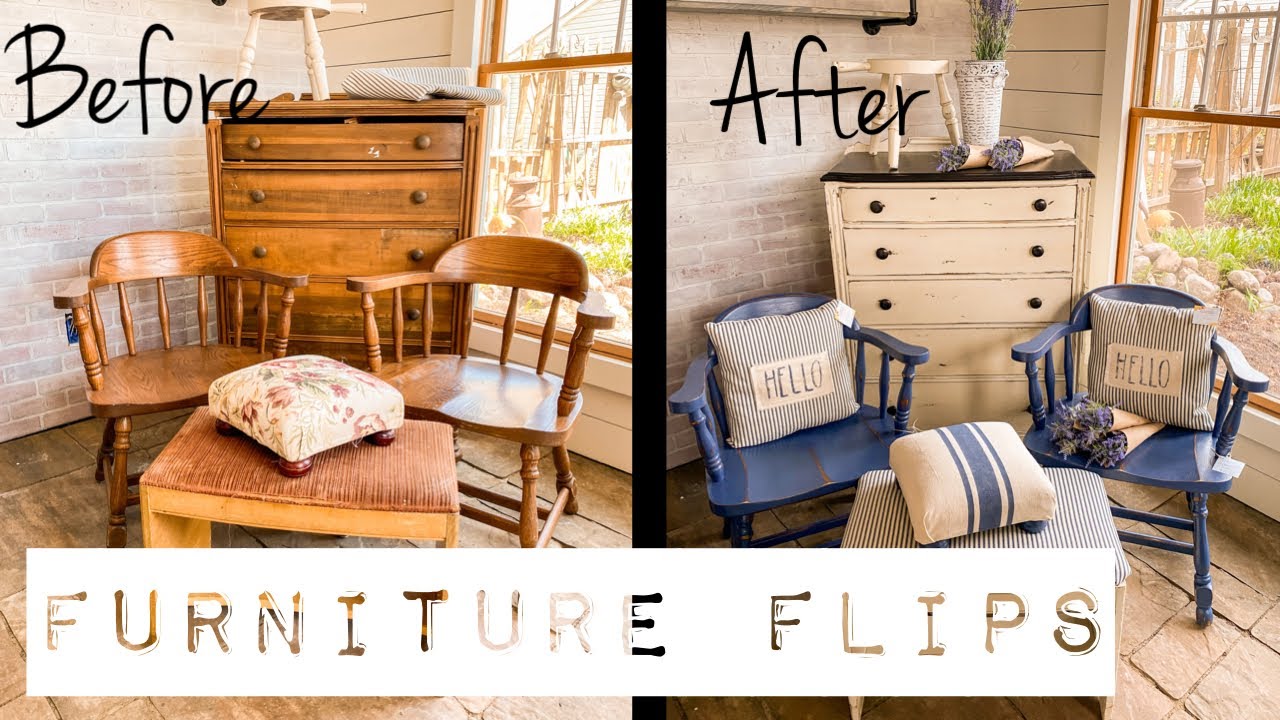This side-by-side image showcases a before and after transformation of a room corner, focusing on a renovation of the same furniture set. Both images, labeled "before" and "after" in black text at the top left corner, depict a section of a house with a white and brownish brick wall, a brown-framed window on the right-hand side, and a stone floor. The "before" picture on the left features a brown dresser, two small brown chairs, a brown ottoman with a floral print, and a small table. In contrast, the "after" picture on the right shows the same furniture pieces that have been updated: the dresser is painted white with a black top, the chairs are now blue with decorative pillows that read "hello," and the ottoman now has a white surface with blue pinstripes. At the bottom, a label on a transparent background reads "furniture flips," indicating the transformation process, with the text allowing the furniture to be seen through it.